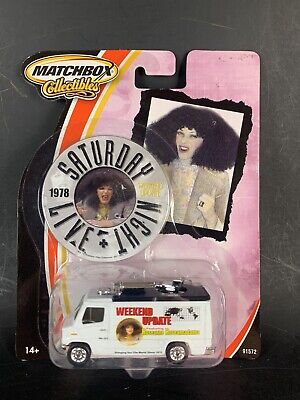The image depicts a Matchbox Collectible toy still encased in its packaging. The toy is a white, rectangular van with black tires and silver hubcaps. On the side of the van, red text reads "Weekend Update." The packaging features a prominent pink background with a black border around certain parts. In the top left corner, there's an oval with a yellow outer rim and a white center, displaying black text that reads "Matchbox," with "Collectables" beneath it in yellow.

A silver circle on the packaging has "Saturday Night Live" written in black text, with "1978" positioned on the left side of the circle. Inside this circle, there is an image of a woman with frizzy black hair. Additionally, a rectangular photo of the same woman, framed in black, is adjacent to the circle. The background includes accents in pink, red, yellow, and white stripes, contributing to the vibrant and themed design that highlights the Saturday Night Live motif. This collectible item seems to be part of a series celebrating the iconic TV show.